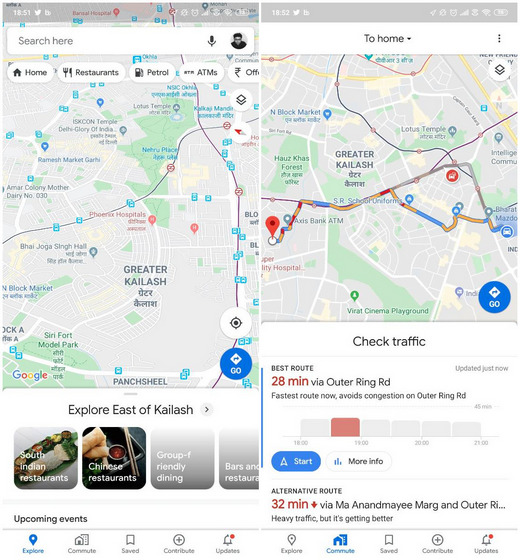In the image, the screen displays someone conducting a search for restaurants using a map application. On the left side of the screen, there is a list of restaurant options including Chinese, South Indian, and group-friendly dining bars. The right side features a navigation menu with filters such as "Home," "Restaurants," "Petrol," and "Offices," suggesting the search is being conducted in a European location. The map page shows a detailed route with an indication to check traffic and a 20-minute travel time via the Outer Ring Road. A secondary map on the side shows directions to return home. The destination indicated is "Greater Kailash," a locality name that does not provide specific context to the user. The image lacks explicit details about the exact destination or origin but clearly outlines the user navigating their route and planning their way back home using Google Maps.